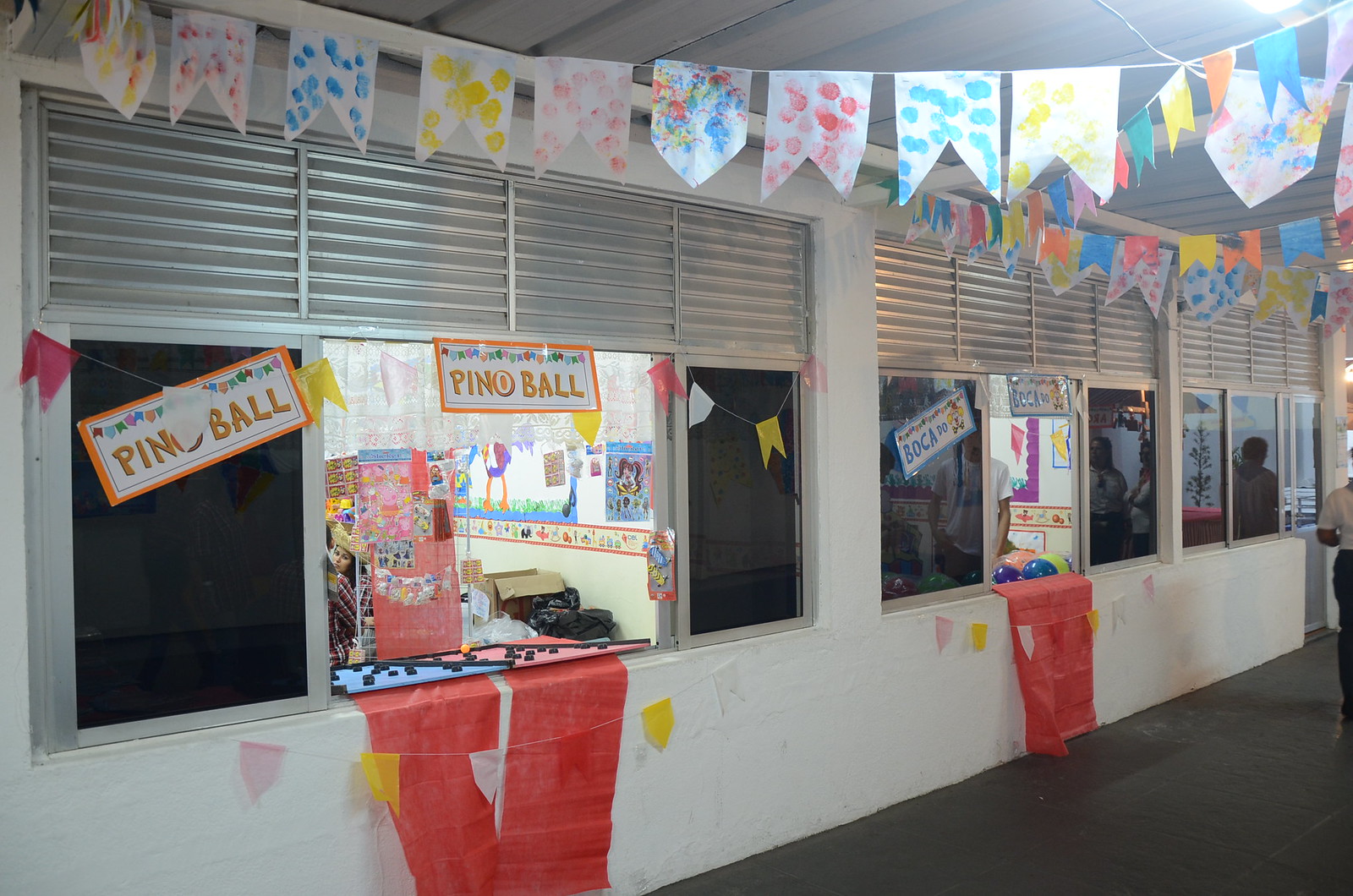The image depicts a festive scene, likely in a school or office setting, characterized by a series of windows adorned with colorful flags and decorations. The white background flags feature vibrant handprints or fingerprints in red, blue, yellow, green, and orange. The right side of the image shows three windows with silver vents; the first and last windows are blacked out, while the middle window is transparent, revealing a person in a white shirt and purple decorations. The walls are white and decorated with various posters and signs in a wide array of colors, including blue, white, yellow, orange, red, purple, pink, and black. One prominent sign reads "Pino Ball" in orange on a white background with an orange outline. The floor appears dark, and there are two red items protruding from both windows. The space is well-lit, suggesting an ongoing celebration or event like “Pino Ball,” with additional flags and balloons in blue, yellow, and purple adding to the festive atmosphere. To the right, a person dressed in a white shirt and black pants is visible, seemingly walking through the area.